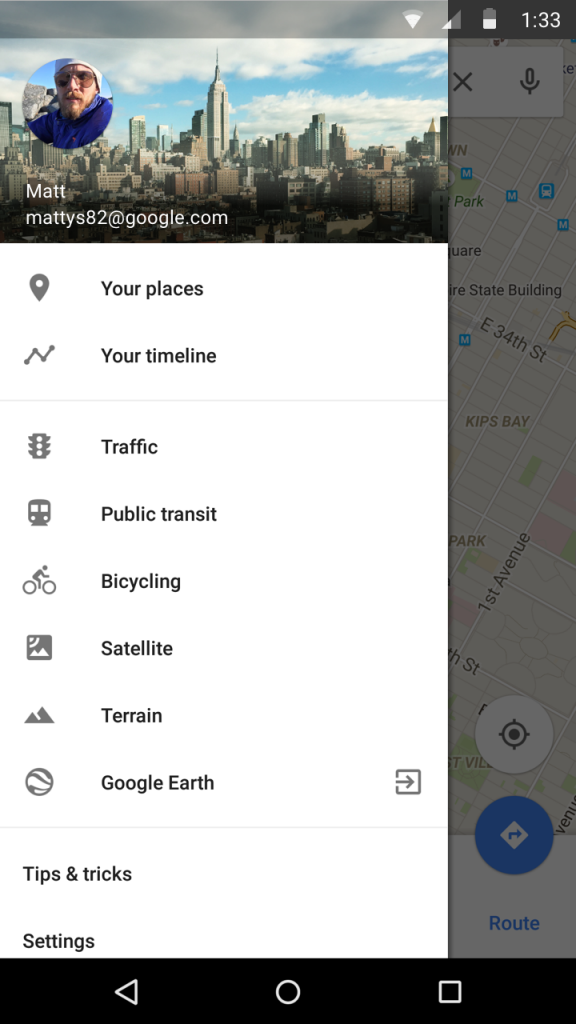Screenshot from a Google Mobile App:

This detailed screenshot appears to be from a mobile version of a Google app, displayed at 1:33 PM with approximately 50% battery life remaining. The interface features two overlapping images: a grayed-out background image of a map and a more prominent foreground image.

The background image showcases a map with visible streets and a highlighted area known as Kips Bay, specifically around 1st Avenue. There are notable icons visible on this map: a white icon and a blue icon, accompanied by the text "route" in blue.

In the foreground, the main focus is on a section displaying an icon of a man with the name "Matt" underneath in white text. Below his name, his Google email address "mattys82 at google.com" is shown. The background of this section features an image of a cityscape with visible skyscrapers against a sky that transitions from blue to white with scattered clouds.

Below this cityscape image, there is a list of selectable options, including:
- Your Places
- Your Timeline
- Traffic
- Public Transit
- Bicycling
- Satellite
- Terrain
- Google Earth
- Tips and Tricks
- Settings

At the bottom of the screenshot, there is a black bar containing three distinct icons, which likely serve as navigation or action buttons for the user.

This composition presents a dynamic and interactive view of a Google app interface, combining mapping features with user-specific information and selectable options, ideal for efficient navigation and personalization.